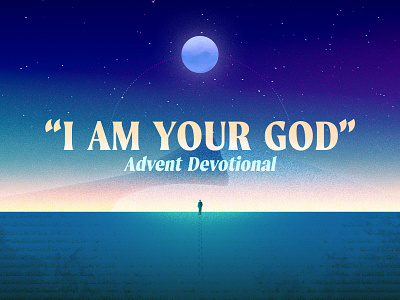The promotional artwork features a surreal, computer-generated scene divided into distinct layers. The sky at the top transitions from a lighter blue at the horizon to a deep, dark blue adorned with scattered white dots symbolizing stars. Dominating the upper center of the image is a blue moon with its lower half shaded darker than the top. 

Beneath this celestial display, the horizon emits a gradient that begins as a soft white and progresses into pinkish and yellowish tones, evoking the subtle light of either dawn or dusk. This horizon meets a semi-transparent blue surface that extends across the bottom of the image, darkening towards the bottom corners. 

At the center of this blue plane stands a solitary black silhouette, possibly male, gazing into the distance. Overlaying the image, in light yellow text, are the words "I am your God," enclosed in quotation marks. Below this, in bold green letters, reads "Advent Devotional," providing the viewer with a clear and serene spiritual message.